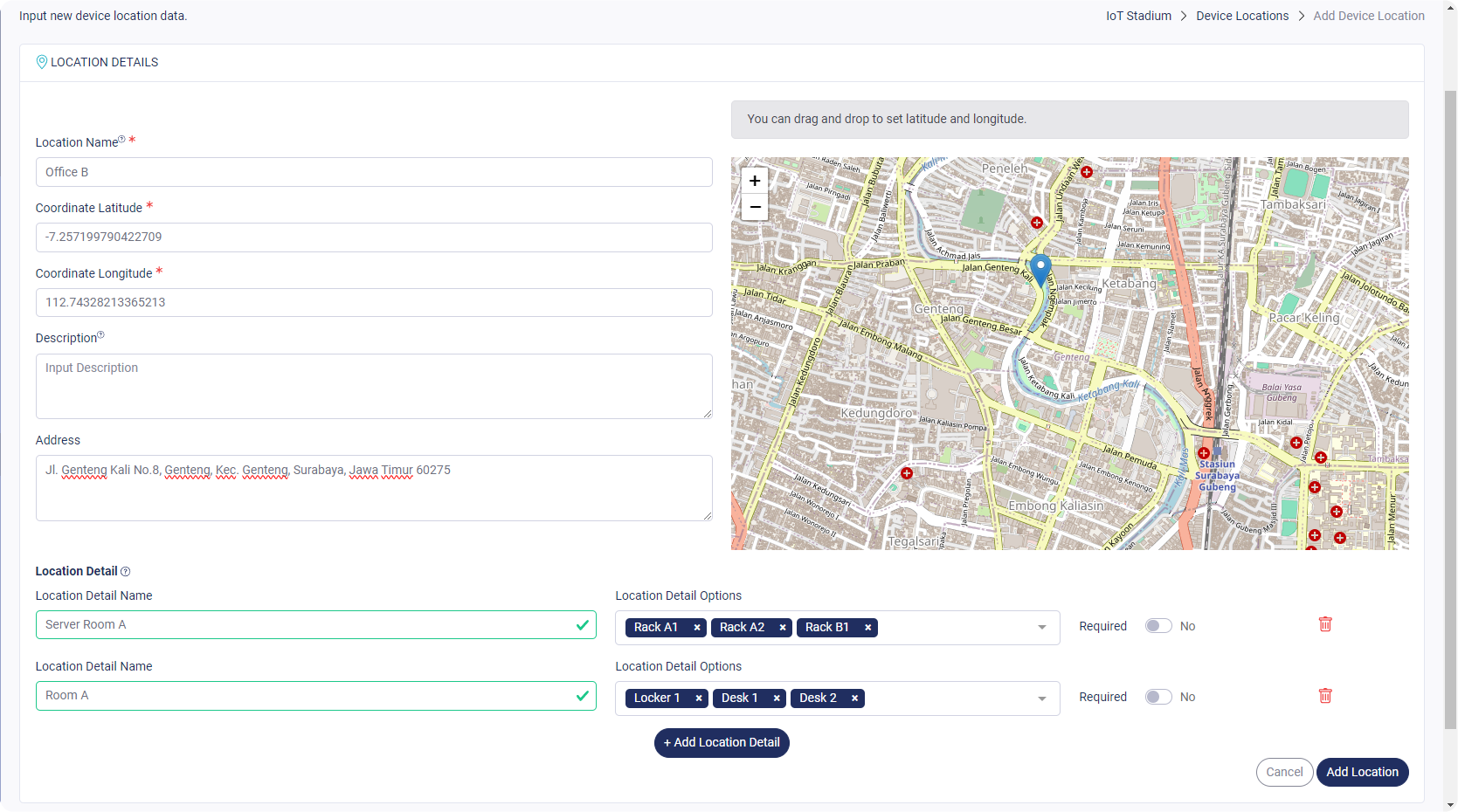This image captures a screen resembling a travel or location management interface, possibly created by Google, though no explicit branding is visible. 

At the top left corner, within a grayish header bar, the text "Input New Device Location Data" is prominently displayed. To its right, a breadcrumb navigation trail reads: "IOT > Stadium > Device > Device Locations > Add Device Location," with each section separated by arrows, the last part in a faded font.

Below this header, on the left side, the section titled "Location Details" features a small icon next to it, likely a location pin. Under this title, the first field labeled "Location Name" includes a red asterisk indicating it is a required field, with "Office B" filled in a long rectangular input box beneath it. Following this are fields for "Coordinate Latitude" and "Coordinate Longitude," each with associated input areas and some faded placeholder or existing data. Adjacent is a section for entering an address, described as "Input Description," again featuring an input box with some data.

In the middle of the screen, two long checkboxes marked with green ticks represent additional location details, though the specifics are not clearly mentioned.

Dominating the center is an integrated map displaying a blue location pin, indicating the specified coordinates. The overall layout suggests a detailed and user-friendly interface for managing or inputting device locations.